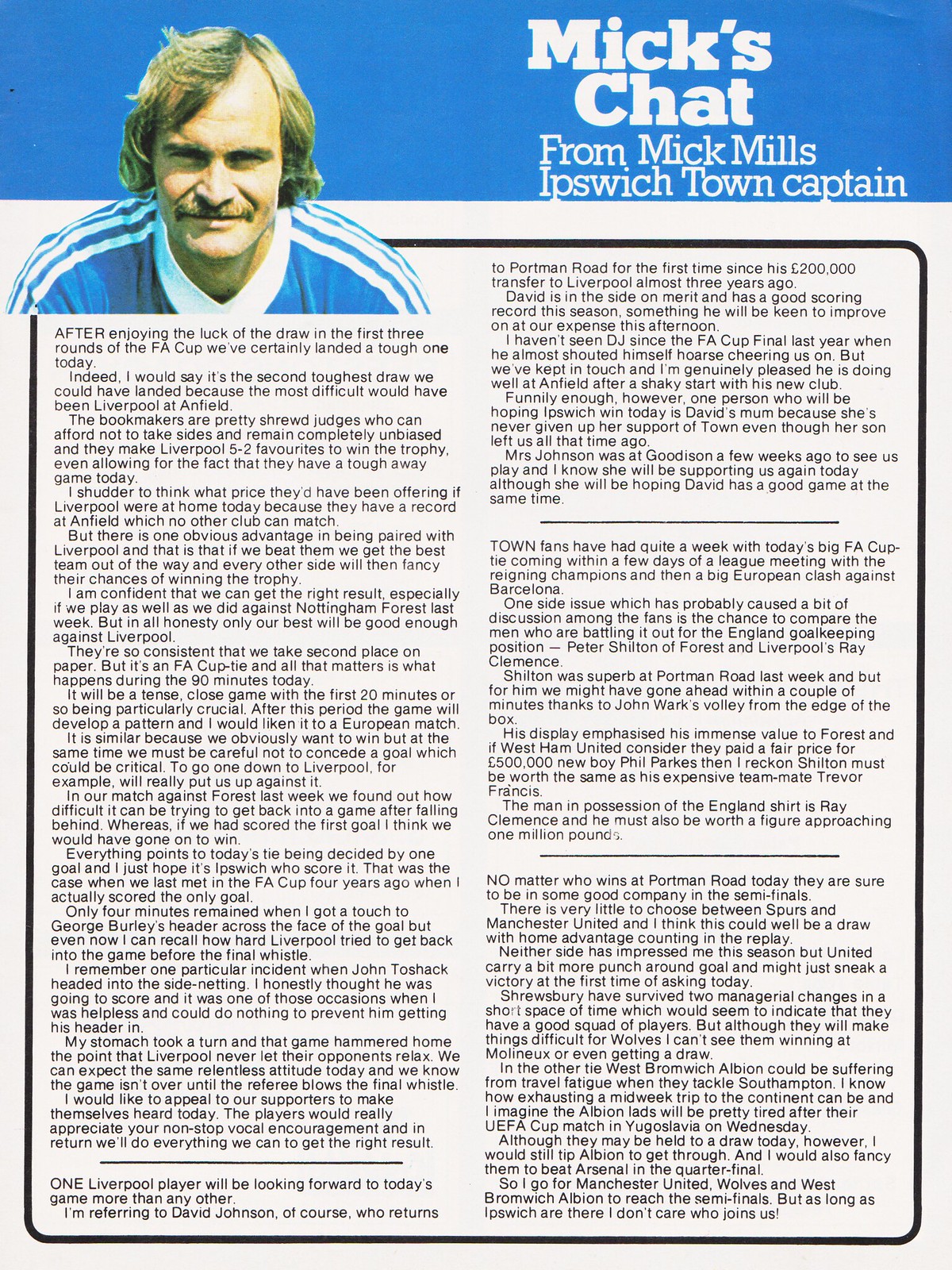This image is a scan of a page from a magazine, a pamphlet, or a program, prominently titled "Mick's Chat from Mick Mills, Ipswich Town Captain." The top of the page features a blue background with white lettering, while the main body of the page is white. To the left, there is a torso-up photo of Mick Mills, who has blonde hair, a large mustache, and is smiling slightly. He is dressed in a blue jersey with white stripes on the shoulders. 

Mick Mills authored the extensive text content on the page, where he discusses Ipswich Town's journey in the FA Cup. After a favorable draw in the first three rounds, they now face a challenging match against Liverpool, which he considers the second toughest draw. Mills elaborates on Liverpool's formidable record at Anfield and how overcoming them would significantly boost their chances for the trophy.

He vividly recalls a previous encounter with Liverpool in the FA Cup, emphasizing the relentless nature of the team and the need for Ipswich Town's supporters to be vocally supportive. He also mentions Liverpool player David Johnson, who transferred from Ipswich three years prior and is expected to perform well, along with his mother, a loyal Ipswich fan.

Mills reflects on recent matches and upcoming challenges, comparing key players like goalkeepers Peter Shilton and Ray Clemence, while expressing confidence in his team's ability to advance to the semi-finals. He makes a final remark on the upcoming oppositions, tipping Manchester United, Wolves, and West Bromwich Albion to join Ipswich Town in the semi-finals. The text is dense and organized into four sections, each at least three to four paragraphs long, showcasing Mick Mills' detailed and passionate commentary on his team's prospects in the FA Cup.